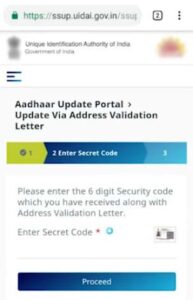The image appears to be a blurry screenshot taken from a mobile device, showcasing a government website, discernible from the URL https://ssup.uidal.gov.in partially visible at the top of the screen. The interface displays two open tabs and includes a hamburger menu for additional options. Directly below the address bar, the website header identifies it as the "Unique Identification Authority of India, Government of India." On either side of this header, there are two indistinct images: one on the left, which appears dark, and another on the right, which has a reddish-yellow hue.

Beneath the header lies a navigational options bar followed by a gray divider line. Below this, the screen is filled with a mix of English and Indian text, displaying a three-step status bar colored in green, dark blue, and light blue. Further down, in a white text box, the website prompts the user to "Please enter the six-digit security code which you have received along with address validation letter." Following this, another instruction to "Enter secret code" is marked with a red asterisk and accompanied by a small green icon, next to an additional indiscernible image. Another gray line follows this section, ending with a prominent blue button labeled "Proceed" in light blue text.